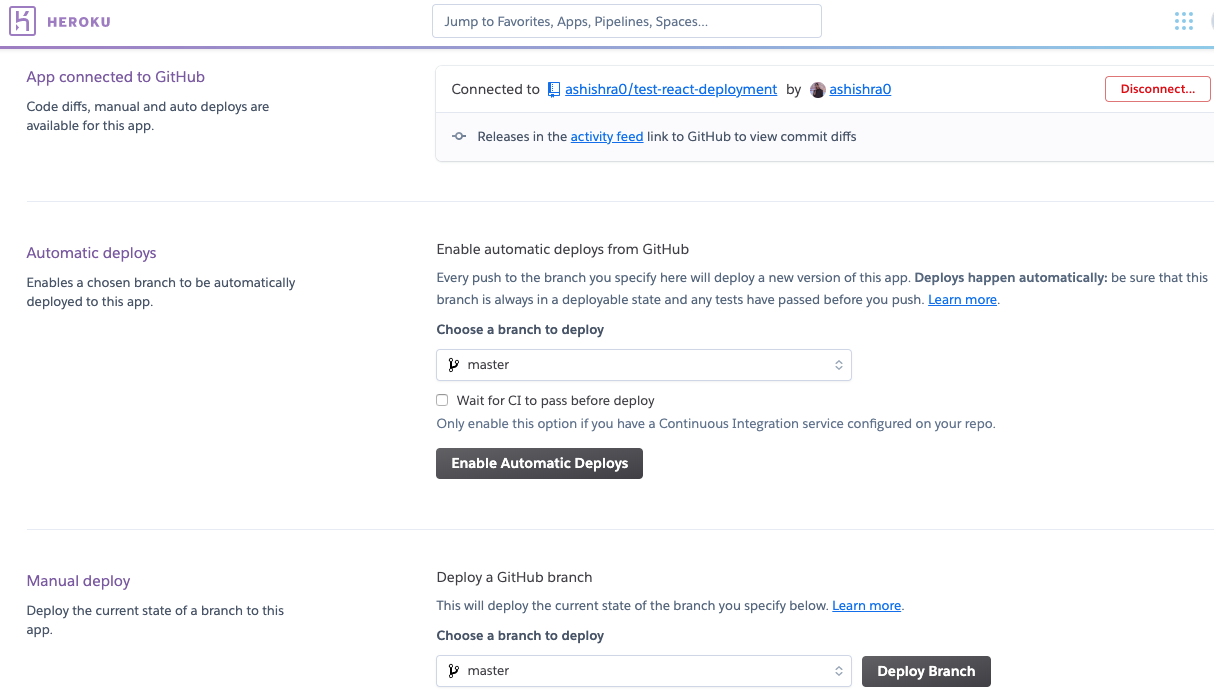This image depicts a Heroku web page interface, primarily used for app deployment and management. On the right side of the interface, there are options and controls organized under categories such as Favorites, Apps, Pipelines, and Spaces. The app shown is connected to a GitHub repository named 'Ashira/test-react-redeployment,' managed by Ashira O.

Features related to the app's deployment are prominently displayed, including both manual and automatic deployment capabilities. The interface indicates that code differences (diffs) can be viewed, and there are settings for both manual and auto-deploys. The app is configured to handle deployments from specific branches, mostly focused on the master branch.

For automatic deployments, the system is set to deploy automatically from GitHub, with an option to enable this feature for the master branch. There is also mention of ensuring the Continuous Integration (CI) tests pass before deploying to maintain a stable state. The interface provides a clear option to initiate a manual deployment, where users can deploy the current state of a specified branch to the app directly. The deployment operations are visually emphasized with black background buttons and white text for ease of visibility and actioning. A 'Deploy Branch' button is provided to facilitate this process.

Additionally, a control to disconnect the app from GitHub is available in the upper right-hand side of the page, indicating the application’s flexibility and user control over integration settings.